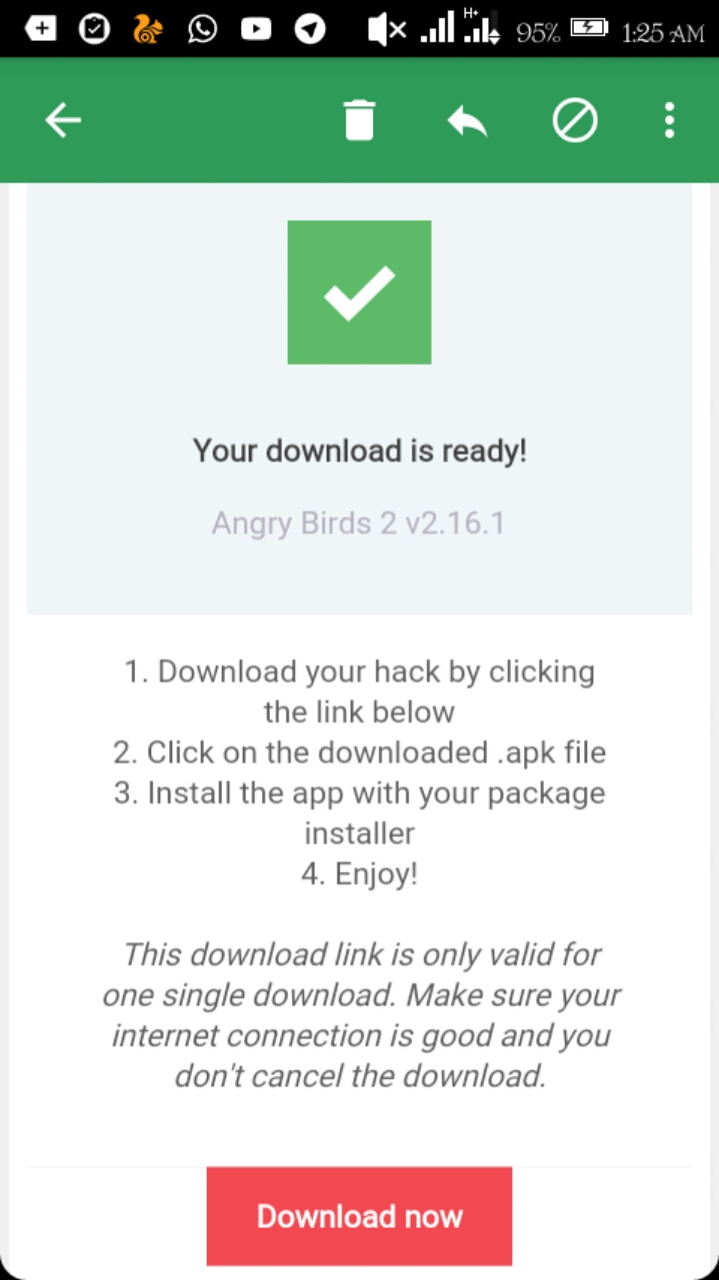The image shows a mobile device, possibly a phone or tablet, in the process of downloading the game Angry Birds. It is 1:25 AM, and the device's battery is at 95% charge. The download is occurring over cellular data, as indicated by the corresponding icons. The sound on the device is muted. 

On the screen, various icons are visible, including:
- A directional arrow
- A play button
- A talk button within a speech bubble
- A squirrel icon in light yellow
- A briefcase with a white checkmark inside a circle
- A thick left arrow with a plus sign

Additional icons below these include:
- A green rectangle with a left-pointing arrow
- A trash bin
- A curved left-pointing arrow
- A white "do not" symbol
- Three ellipses

At the bottom, there is a gray box containing a green rectangle with a white checkmark and the message, "Your download is ready. Angry Birds 2 version 2.16.1."

Following these icons and messages, the background is predominantly white, displaying instructions for using a downloaded hack. The steps provided are:

1. Download your hack by clicking the link below.
2. Click on the downloaded APK file.
3. Install the app with your package installer.
4. Enjoy.

It’s also noted that the download link is valid for a single use only and warns to ensure a stable internet connection without canceling the download. A prominent red button labeled "Download Now" is present at the bottom of the screen.